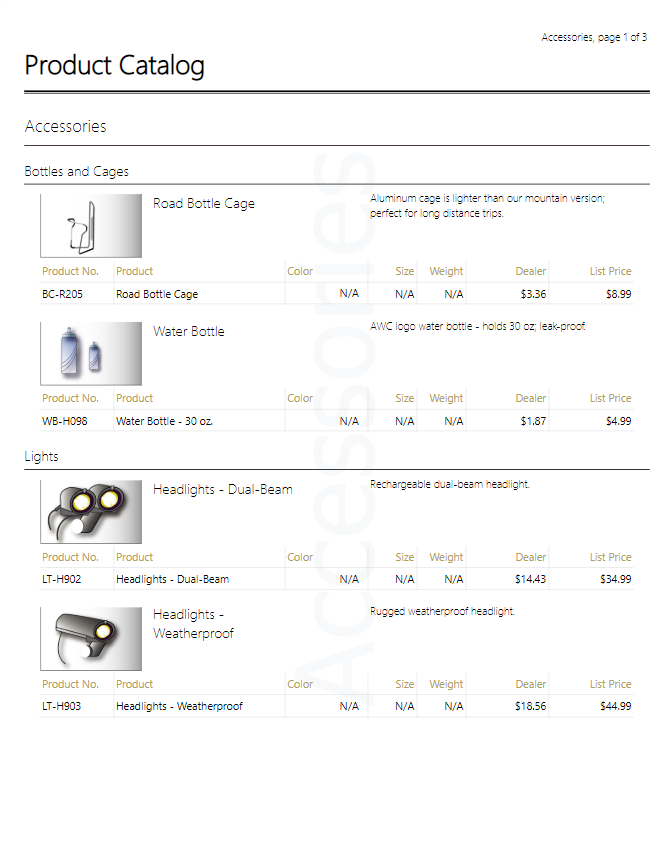Here is a detailed and cleaned-up caption for the image based on the provided description:

---

This image showcases a section of a product catalog, specifically focusing on accessories, as indicated by "Accessories, Page 1 of 3" in the top right-hand corner. The catalog page is titled "Product Catalog," and features subcategories "Accessories" and "Bottles and Cages."

Highlighted products include:

1. **Road Bottle Cage**:
    - Description: Aluminum cage, lighter than the mountain version, ideal for long-distance trips.
    - Dealer Price: $3.36
    - List Price: $8.99

2. **AWC Logo Water Bottle**:
    - Description: Holds 30 ounces, leak-proof design.
    - Dealer Price: $1.87
    - List Price: $4.99

3. **Dual Beam Headlights**:
    - Description: Rechargeable dual beam headlights.
    - Dealer Price: $14.43
    - List Price: $34.99

4. **Rugged Weatherproof Headlights**:
    - Description: Durable and weatherproof construction.
    - Dealer Price: $18.56
    - List Price: $44.99

This catalog page provides detailed pricing and product descriptions, highlighting potential profit margins for dealers.

---